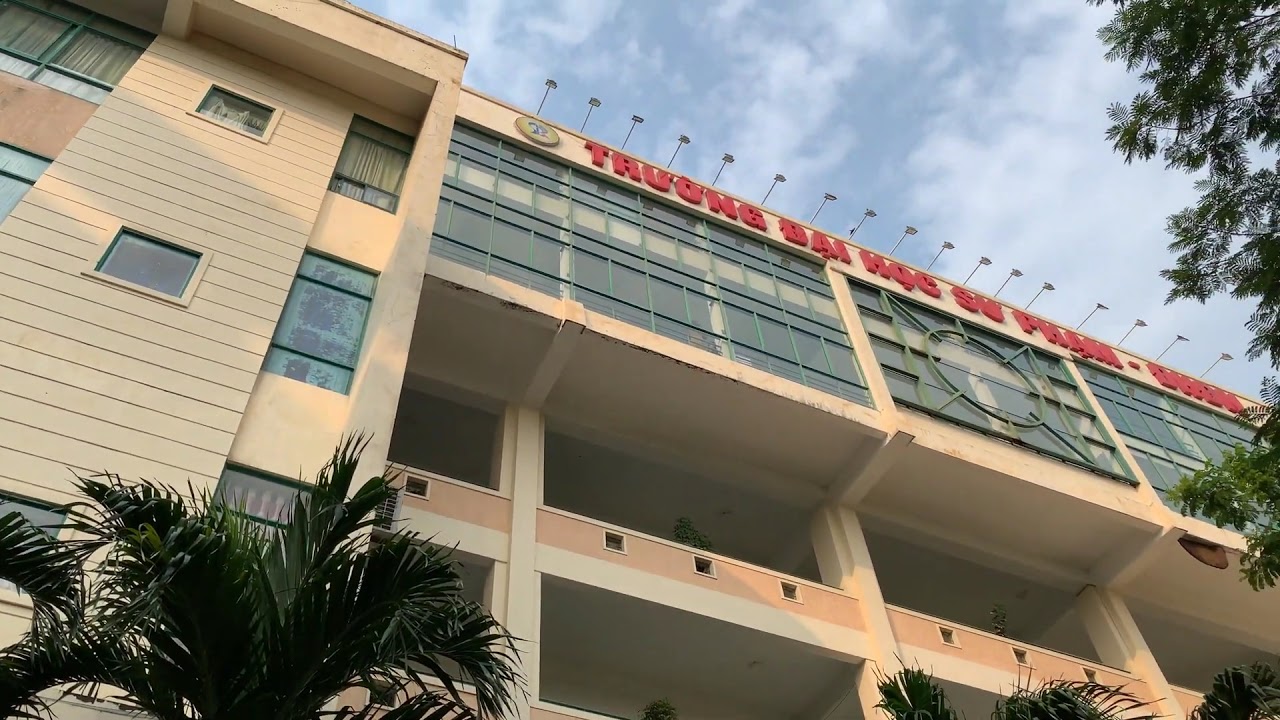This image captures an upward view of the University of Da Nang in Vietnam, emphasizing the building's grand exterior. The structure, adorned with large red Vietnamese lettering at the top, spells out "Truong Dai Hoc" and features a circular emblem on the left. The top of the building is equipped with metal bars hosting lights that illuminate the façade, enhancing its stadium-like appearance. Beneath the signage are expansive windows, possibly indicating multi-story levels with open segments resembling a parking garage. The building's exterior showcases a beige and white palette and boasts numerous balconies, some adorned with plants. The foreground is lush with palm trees and additional greenery to the right, set against a backdrop of a blue sky with scattered white clouds.